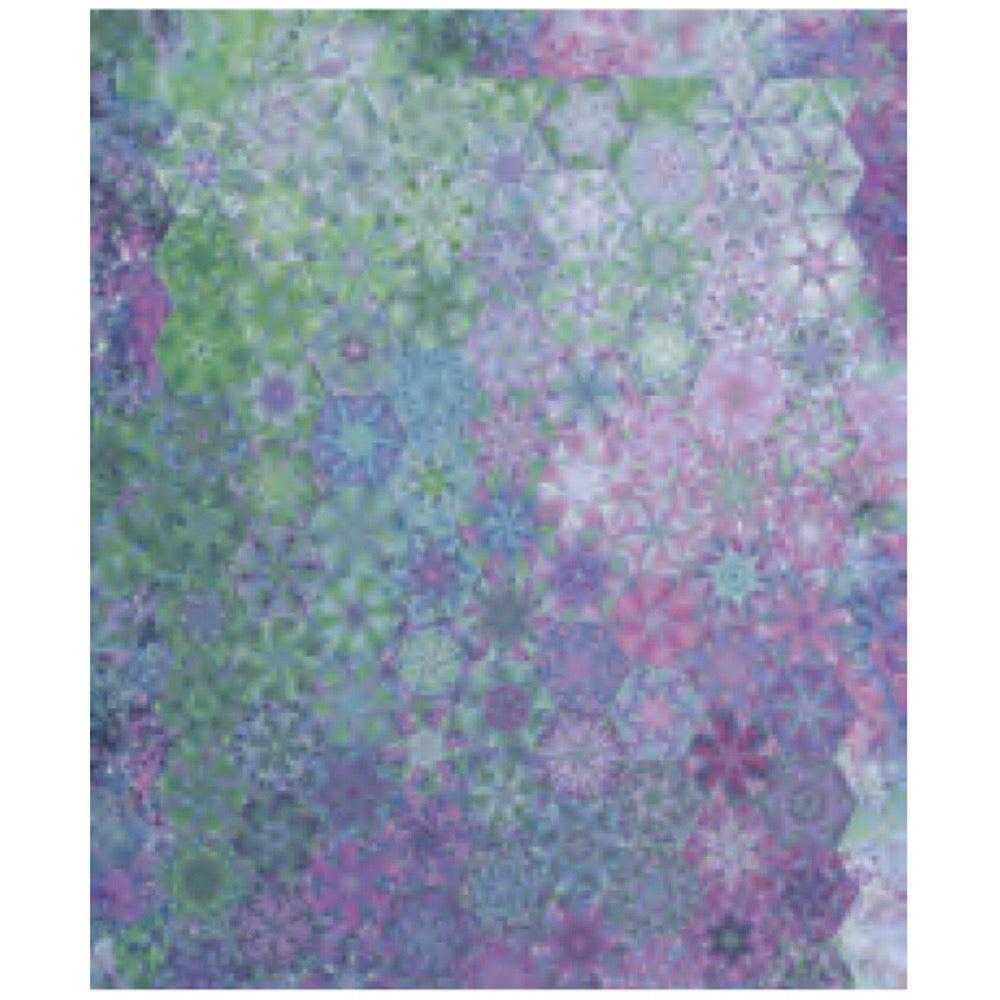The image is a mesmerizing, kaleidoscopic composition dominated by numerous hexagonal shapes, creating an intricate, abstract pattern. Each transparent hexagon is filled with a snowflake-like, star, or floral design, and the array of colors ranges across vibrant greens, blues, purples, and pinks, interspersed with shades of red. The hexagons are meticulously arranged, covering the entire frame, and the background complements the shapes with a blur of the same colorful palette. It evokes the feel of a magnified view of a decorative panel, perhaps a painting or digital artwork, evoking thoughts of tile work or a sophisticated art piece, although the specific context remains unclear. This visually stunning image lacks textual elements, drawing the viewer's attention solely to its vivid and complex geometric beauty.